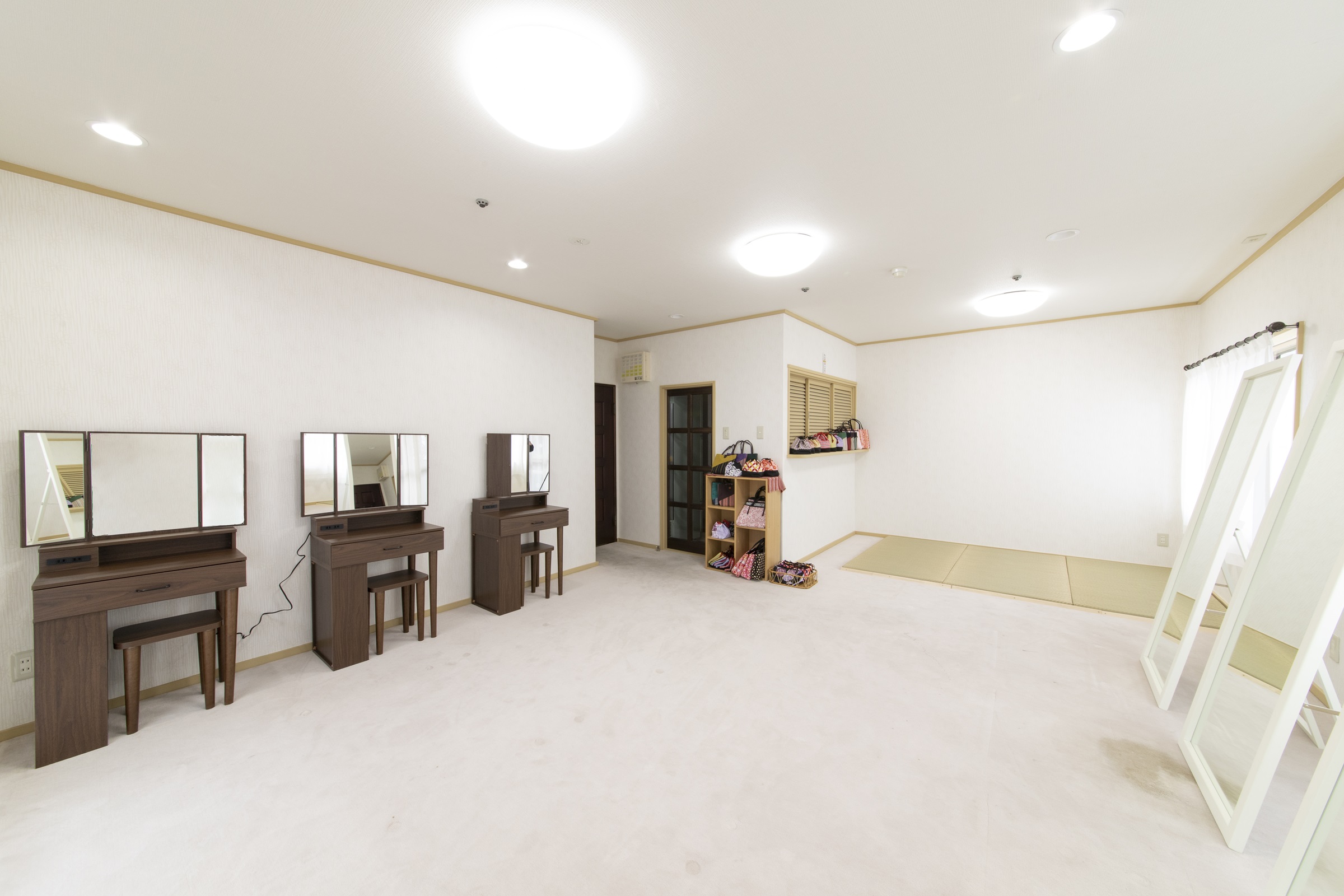The image depicts a large, pristine, and well-lit room that appears to serve as a dressing or changing room, possibly within a house, basement, or studio apartment. The entire space exudes a predominantly white color scheme, featuring white carpets, walls, and ceiling. The ceiling is adorned with bright recessed circular lights, contributing to the room's radiant illumination. 

On the left side of the room, three brown wooden dressing tables are positioned against the wall. Each table is equipped with a long drawer and has a short stool tucked underneath. Atop each table sits a three-fold mirror, enabling a complete view for users seated at the tables. 

On the opposite side, the right-hand wall showcases three large, full-length mirrors with elegant white frames, each standing on the floor. Towards the upper right corner of the image, there is a window dressed with white curtains and a section of the floor is covered in tile. Notably, the room's furnishings and objects are scattered rather than centered, adding to the impression of an expansive, open space. A brown trim or crown molding subtly accents the ceiling, adding a touch of sophistication to the room's overall aesthetic. The absence of text in the image keeps the focus on the detailed arrangement and cleanliness of the space, with colors including white, brown, tan, pink, red, blue, black, and silver appearing throughout the room.